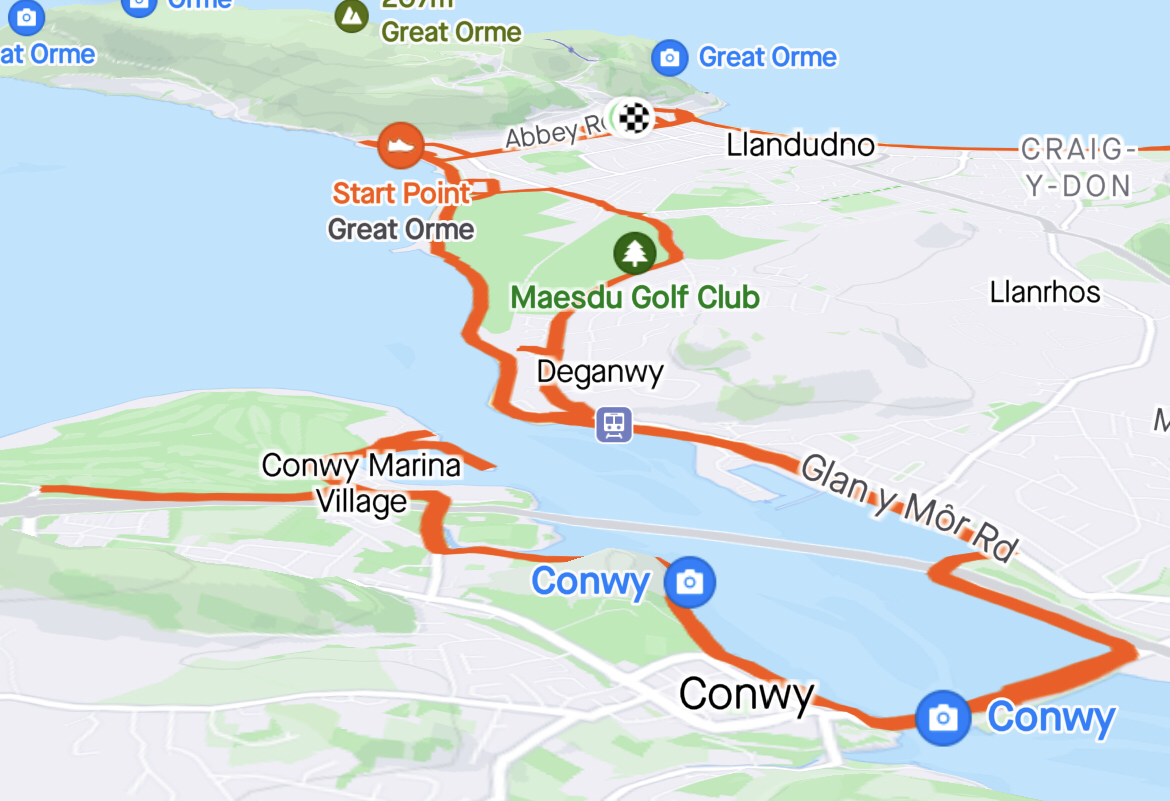This computer-generated map depicts a horizontal rectangular section showcasing a coastal region with various landmarks and routes. On the top left, the land mass labeled "GREAT ORME" in black lettering outlined in white stands out, bordered by green areas indicating forests and blue sections representing waterways. The map highlights several key locations using symbols, including blue circles with white cameras next to names like "GREAT ORME" and "CONWAY".

A prominent orange path, marked as a potential driving or walking route, starts at a "start point" at the bottom left corner labeled "CONWAY MARINA VILLAGE". It winds through notable areas including "GLAN Y MORE ROAD", and continues upward. Important landmarks along this route include "DAGENY" near a train station symbol, "MAESDU Golf Club" indicated by a tree symbol, and the coastal town "LLANDUDNO" marked in black letters. The route eventually circles back, encountering a bridge labeled "CONWAY" before concluding at a checkered flag near "ABBEY".

Additionally, the map features other names and locations such as "CRAIG Y DON" and "LANRHOS", providing a detailed view of the area with clearly marked roads, paths, and key attractions. The intricate layout of roads and points of interest suggests a detailed guide potentially designed for travelers or explorers.